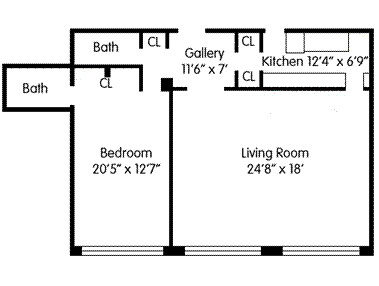This is a detailed photograph of a blueprint drawing, depicting the layout of one floor of a house. Upon entering through the front door, you are greeted by a gallery measuring 11 feet 6 inches by 7 feet. Two closets line the gallery. Proceeding to the right from the entrance, you encounter a hallway leading to a bathroom and a closet. Adjacent to these is a spacious bedroom, boasting dimensions of 20 feet 5 inches by 12 feet 7 inches. This bedroom includes two closets and an en-suite bathroom.

Directly opposite the entrance, at the end of the gallery, you are welcomed into an extraordinarily large living room, which measures a vast 24 feet 8 inches by 18 feet. This expansive area stands in stark contrast to the significantly smaller kitchen, accessible from the living room. The kitchen's dimensions are a cramped 12 feet 4 inches by 6 feet 9 inches, rendering the space barely sufficient for comfortable movement. This disparity highlights the peculiar architectural design, featuring a substantial living room paired with an undersized kitchen.